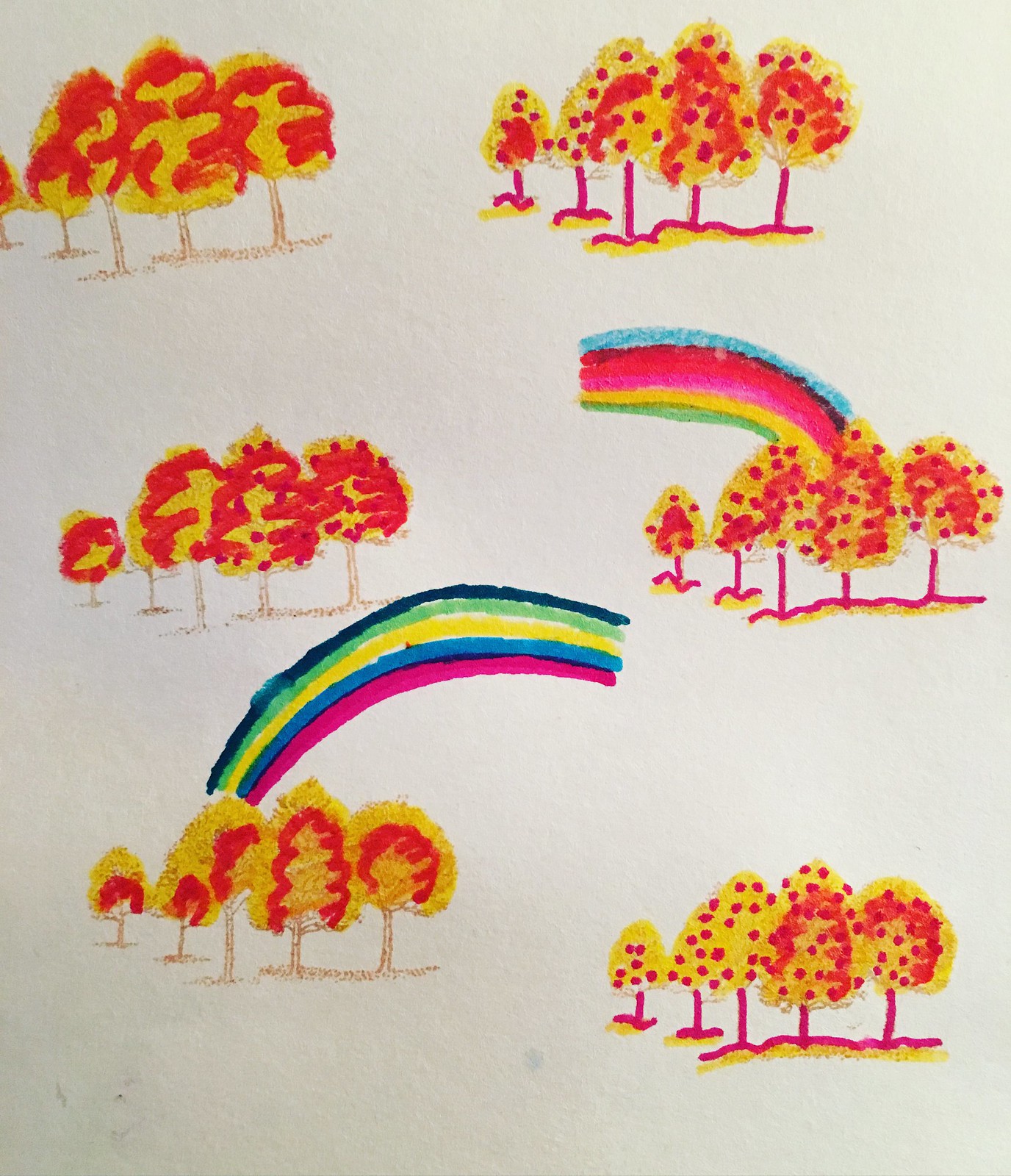This photograph depicts an artistic drawing, potentially derived from a coloring book or a decorated sheet of fabric, meticulously colored with markers. The artwork showcases several groups of fall trees, resplendent in their seasonal foliage of vibrant reds, oranges, and yellows. Some trees are adorned with what appear to be red apples, adding a touch of charming detail to the scene. In the background of two tree clusters, there are rainbows arching through the sky—one exhibiting an array of dark green, light green, yellow, blue, and red, while the other showcases shades of blue, red, pink, yellow, and green. The repeated patterns of the trees and rainbows suggest a theme of autumnal beauty and simplicity, underscored by the consistent and intricate coloring work done with markers.